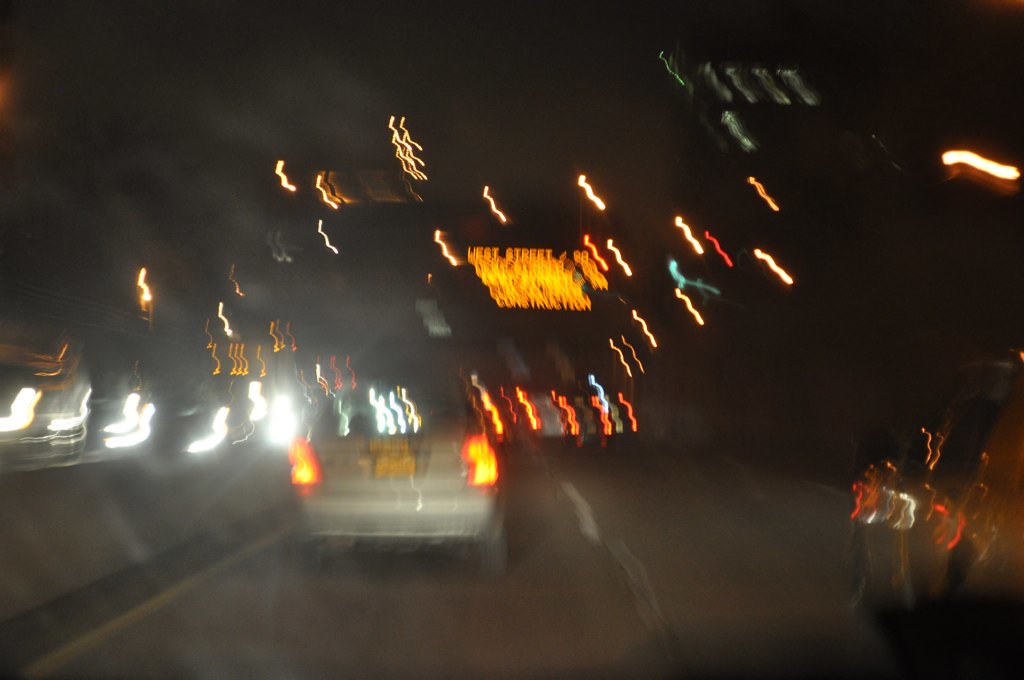Captured from the inside of a moving car, this photograph offers a blurred, dynamic portrayal of a busy highway scene at night. Taken through the windshield, the image foregrounds a silver car immediately ahead and another vehicle traveling alongside. Opposite the direction of travel, a seemingly endless row of headlights advances, contributing to the sense of bustling activity. The road is illuminated by multicolored lights—red, green, and yellow—suggesting traffic signals and signage, all stretched into elongated streaks due to the motion. The overall effect is a chaotic yet captivating display of urban life in perpetual motion.